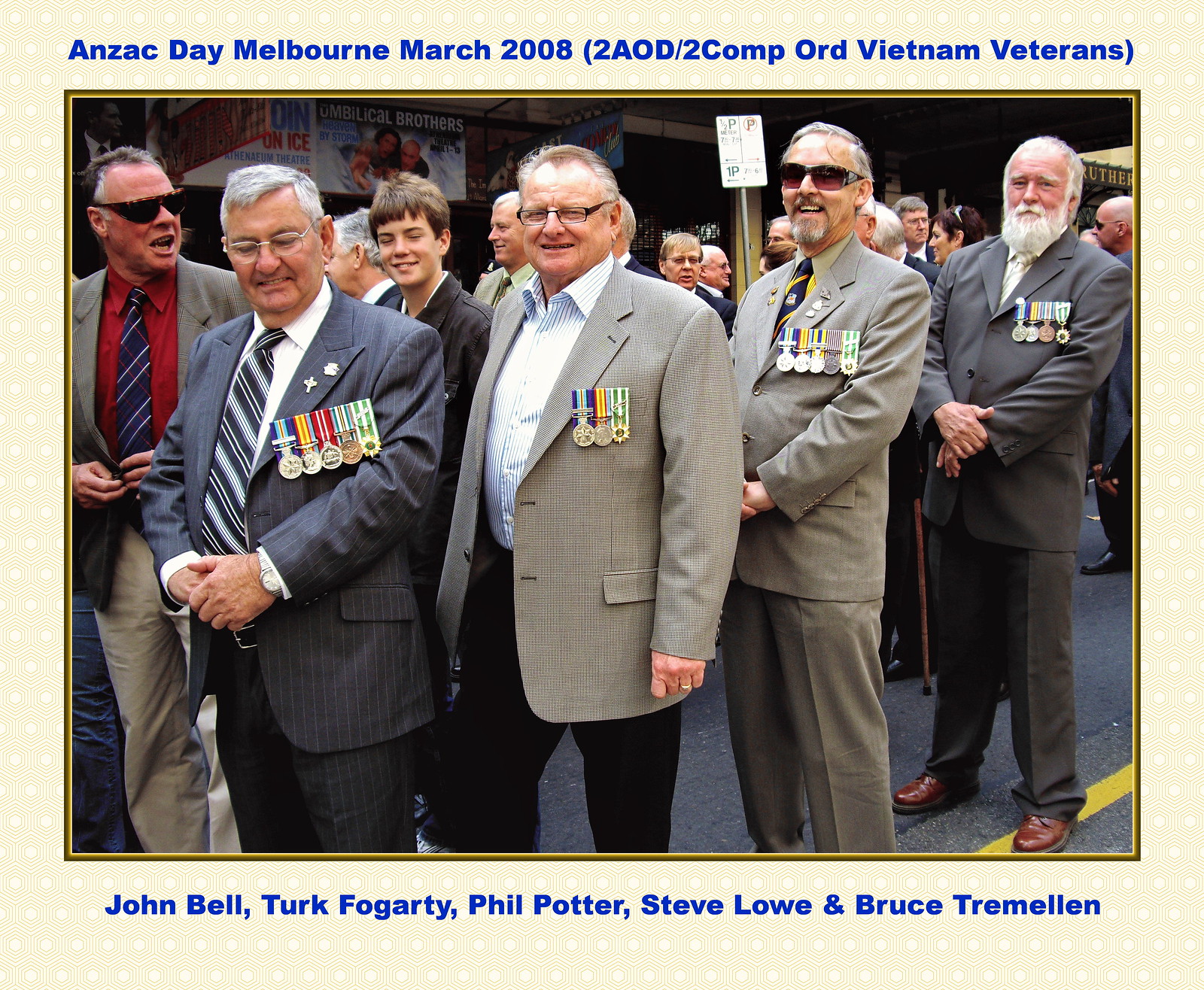This image captures a solemn yet celebratory moment from Anzac Day in Melbourne, March 2008, featuring Vietnam veterans from Australia. Prominently displayed at the top of the photo is the title, "Anzac Day, Melbourne, March 2008," followed by the notation "(2AOD/2COMP, Board Vietnam veterans)." In the front row, a group of older men, likely in their 60s or early 70s, march with a dignified air, each wearing suit or sports jackets adorned with numerous medals on their left lapels, a testament to their service. 

The veterans identified in the caption below the image include John Bell, Turk Fogarty, Phil Potter, Steve Lowe, and Bruce Tremellin. John Bell is particularly noted for his gray jacket paired with a red shirt, blue tie, and khaki pants, along with sunglasses shielding his eyes. Other men in the front row showcase a variety of attires — from gray suits with blue and white striped ties to light brown suits with blue and orange striped ties, all proudly displaying their medals.

A young boy can be seen marching with them in the top left, symbolizing the bridge between generations. The street's yellow center line is visible in the lower right, grounding the procession in an urban setting. Behind these veterans, younger people, possibly their descendants, walk along, smiling and cheering them on, adding to the camaraderie and respect evident in the scene. Spectators line the background, reflecting on the parade and the legacy of those who served.